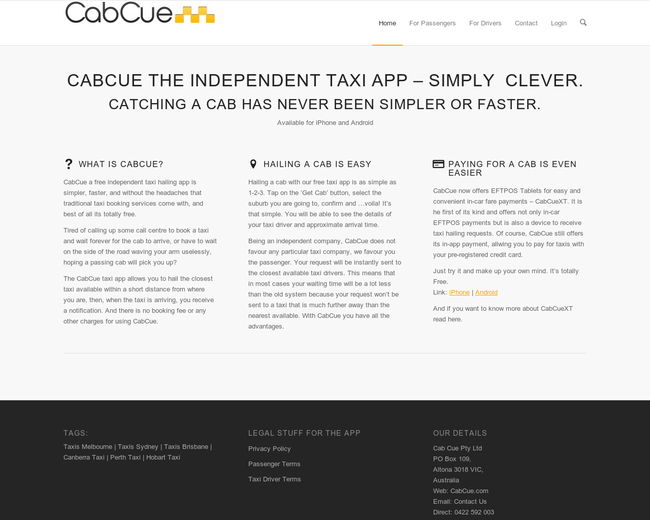The image is a screen capture of a website for an independent taxi hailing app named CabQ, prominently displayed in the top left corner along with its logo, which consists of three yellow boxes stacked on top of one another with additional yellow boxes underneath, resembling a chessboard pattern. The website's headline, "CabQ, the independent taxi app: Simply clever," promises that catching a cab has never been simpler or faster. The layout of the webpage is divided into three main sections, each with its own descriptive heading: "What is CabQ?" on the left, "Hailing a Cab is Easy" in the center, and "Paying for a Cab is Even Easier" on the right. Each section elaborates on the features and ease of use of the app, including that it's free, available for both iPhone and Android, and eliminates traditional taxi booking headaches. Along the top right, there are menu options such as Home for Passengers, For Drivers, Contact, Login, and a magnifying glass icon for search. At the bottom of the page is a black border containing legal information, contact details including a P.O. box, phone number, email, and a site map.